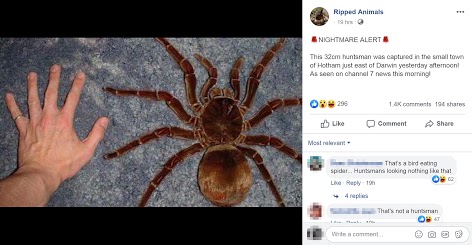The image depicts a striking and somewhat alarming scene. Set against a backdrop framed by black bars at the top and bottom and blue carpet-like texture on either side, a human hand is placed flat on a rock in the center. The hand, extending just a bit past the wrist, shares the frame with an imposing tarantula on the right side. 

The tarantula, which appears lifelike but exaggeratedly large, is approximately twice the size of the hand. The spider's body, consisting of a head and thorax, is about the same size as the palm of the hand, while its legs project outward making it seem much larger. The tarantula features two prominent eyes and what appear to be antennae, giving a stark detail to its intimidating presence. 

Adding to the dramatic effect, the right side of the image has text stating: "Ripped animals nightmare alert: This 32-centimeter Huntsman was captured in a small town of Hotham in the east of Darwin yesterday. As seen on Channel 7 news this morning." Accompanying the text are various social media engagement metrics, including 206 emojis, 101.4 thousand comments, and 194 shares. The commonly seen social media options for liking, commenting, and sharing are also present, suggesting this is a screenshot of a post that has attracted significant attention.